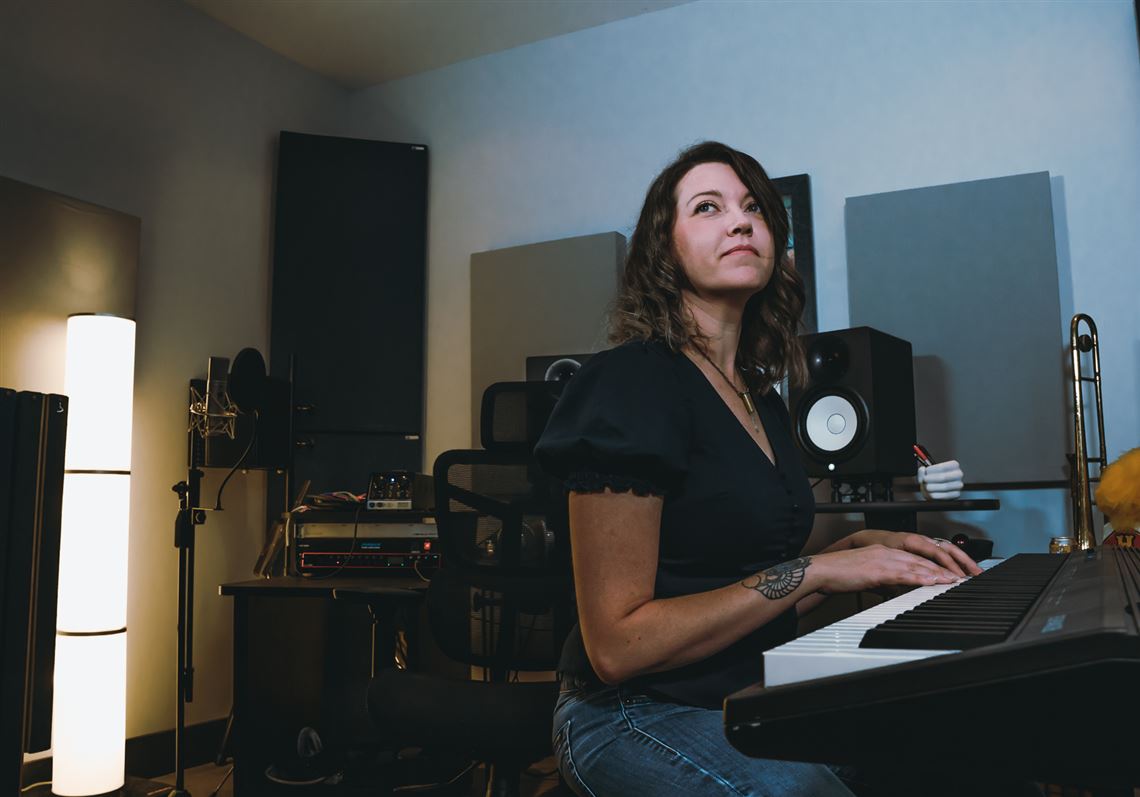In the image, a woman with wavy, chestnut brown hair styled with a slight swoop sits in a recording studio. She wears a black puff sleeve shirt, jeans, and a necklace. Her hands rest on the white keys of a keyboard in front of her, revealing a tattoo on her upper arm. The woman gazes off into the distance to the left, appearing thoughtful. Behind her, various pieces of audio equipment are visible, including black speakers and a tall microphone on a stand fitted with a pop filter. A light stands three feet high in the corner, casting a subtle glow. Additionally, the top part of a brass instrument, possibly a trumpet, is seen, contributing to the studio’s musical ambiance. Although she is seated at the keyboard, she isn't looking at it, suggesting a moment of distraction or contemplation.